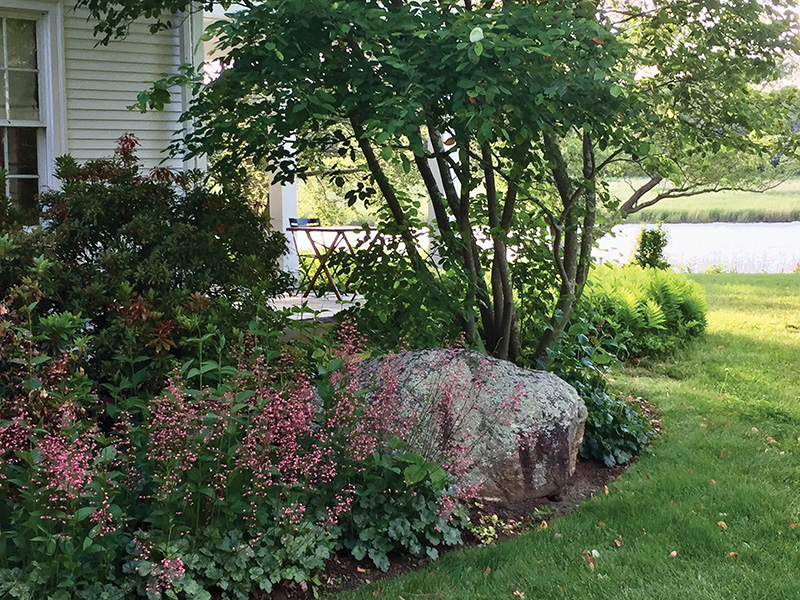This contemporary photograph captures a charming yard in a well-maintained neighborhood. The centerpiece is a large, smooth boulder adorned with a variety of pink flowers and deep green foliage, some of which cascade over the rock. To the right stands a relatively tall tree, possibly a crepe myrtle, with visible branches and an umbrella-like canopy of leaves. The yard features lush green grass and a tidy flat lawn extending to the right. In the background, partially obscured by greenery, is a street with grass on either side, suggesting a pleasant neighborhood ambiance.

On the left side of the image, a small garden showcases additional greenery and tall pink flowers. You can also catch a glimpse of the house, which has cladrood or light cream siding with white trim, and a small portion of a window. A quaint porch is visible with a small table and folding chair, adding to the cozy atmosphere. Beyond the yard is a body of water, possibly a pond or lake, with more trees and greenery in the distance, enhancing the picturesque setting. The overall scene combines natural beauty with a touch of domestic charm, making for a serene and inviting outdoor space.